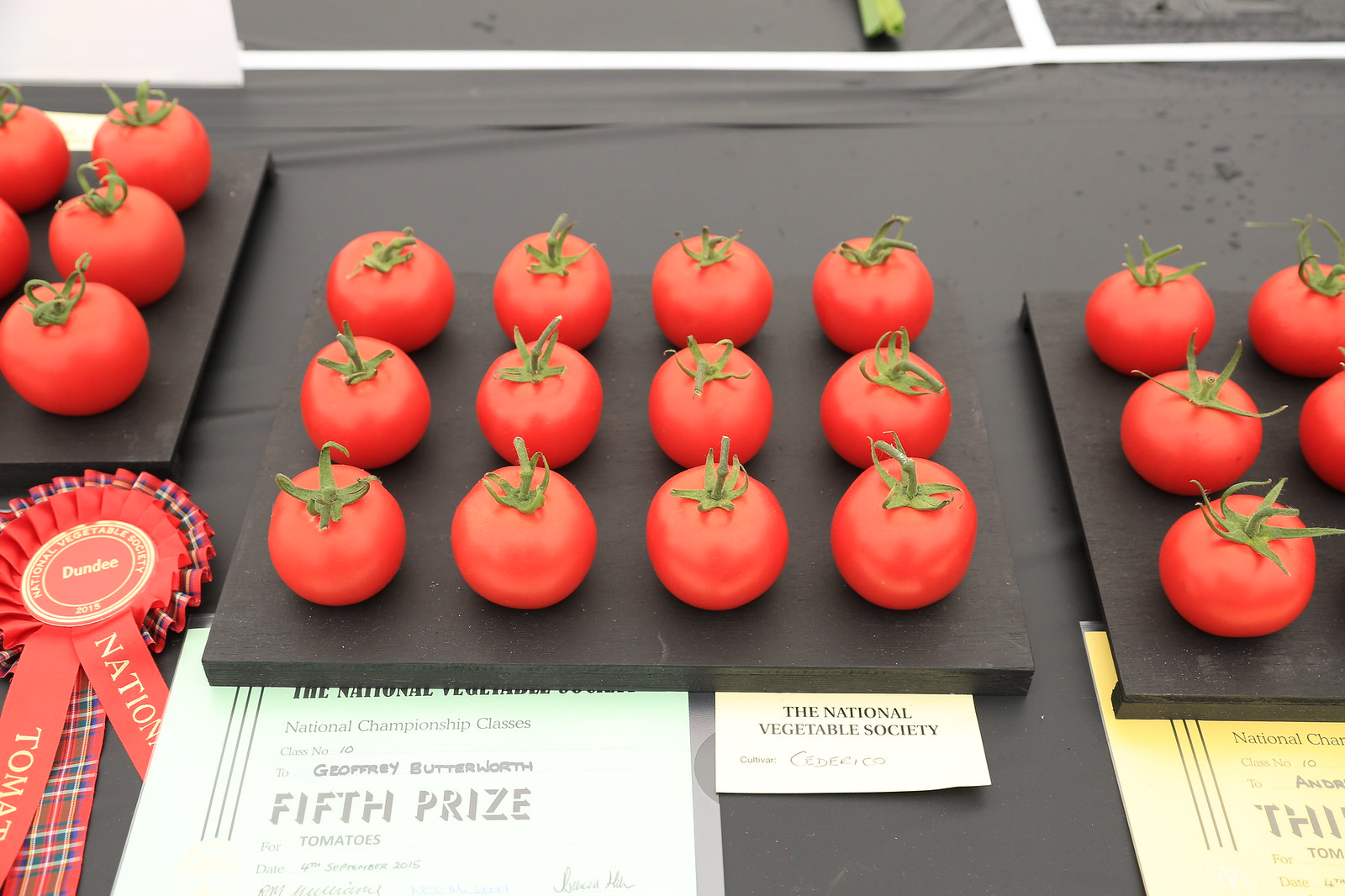In this rectangular image, several bright red tomatoes with pointy green leaves at their tips are meticulously arranged on a black wooden board at the center, forming three neat rows of four. This board is placed on a smooth-looking black material that covers the table. To the left and right in the background, you catch a glimpse of additional platforms, each displaying at least five more tomatoes, though their full extent is cut off by the edges of the image.

Prominently featured in the bottom left corner is a decorative ribbon topped with a wreath, accompanied by flat ribbons cascading down. A broad green paper labeled "Fifth Prize" is also visible. Further details reveal that this accolade was awarded by the National Vegetable Society, with Jeffrey Butterworth as the recipient for his entry in the National Championship Classes. The date marked on the card is September 4th, 2015. The tomatoes, fresh and vibrant with dark green stems, showcase the care and precision put into their presentation for this food contest.